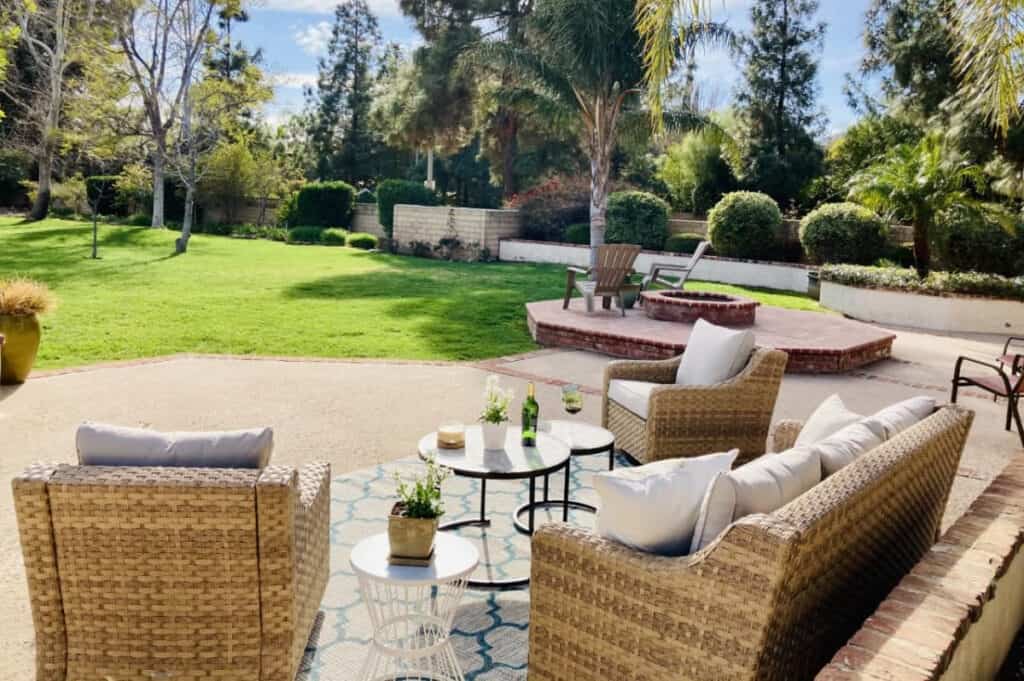This horizontal image showcases an advertisement for outdoor furniture, featuring an inviting arrangement of woven wicker sofas and chairs in brown and tan hues with light gray cushions. Central to the composition is a three-sectioned sofa situated against a brick wall, which features a mix of low and high sections, painted white in parts. This setup overlooks a meticulously manicured lawn adorned with a scattering of trees. A prominent large urn-like planter filled with light yellowish plants adds a touch of elegance to the scene.

In the foreground, two small round tables complement the furniture. One table holds a bottle that appears to be wine and a small white vase containing tall white flowers. Another round table, distinctive for its white open wire basket frame, sits on top of a carpet beneath the seating area and also features a potted plant.

The backdrop is completed by a vibrant blue sky dotted with fluffy white cumulus clouds, enhancing the serene and picturesque quality of this outdoor setting.